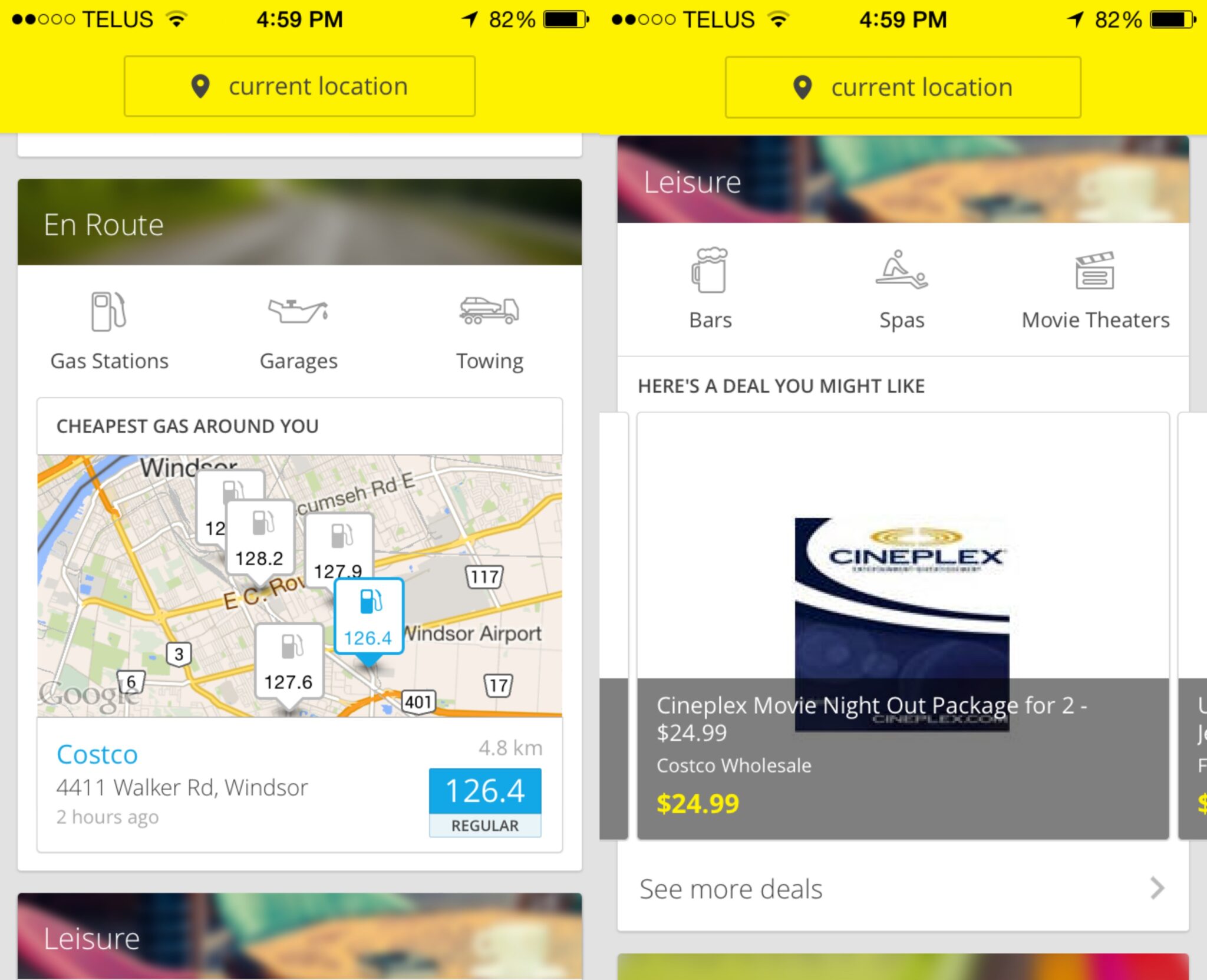The image is divided into multiple sections, each offering different types of information. 

At the top of the image, there's a long yellow rectangle serving as the background. Within this section, there are two out of five circles filled in black. Next to these circles, the word "TELUS" is prominently displayed in uppercase letters. The time is shown as 4:59 PM, with the battery life indicated at 82 percent.

On the left side of the image, the word "ENROUTE" is written in bold, uppercase letters. Below this, several icons and corresponding labels are listed: a gas pump icon followed by "Gas Stations," a symbol depicting liquid pouring from a spout labeled "Garages," and an icon of a car on top of a truck with the label "Towing." Additionally, there is a note stating "Cheapest gas around U," accompanied by squares indicating the distances to various gas stations.

One of the gas stations listed is Costco, located at 4411 Walker Road, Windsor. This information is highlighted within a blue rectangle displaying "126.4," and it is noted to be 4.8 kilometers away.

On the right side of the image, under the section labeled "LEISURE," are options for "Bars," "Spas," and "Movie Theaters." Centrally placed within a navy blue and white square, the word "CINEPLEX" is prominently displayed. Beneath this, a description reads "CINEPLEX Movie Night Out, package for two, $24.99," with the phrase "Costco Wholesale $24.99" highlighted in yellow.